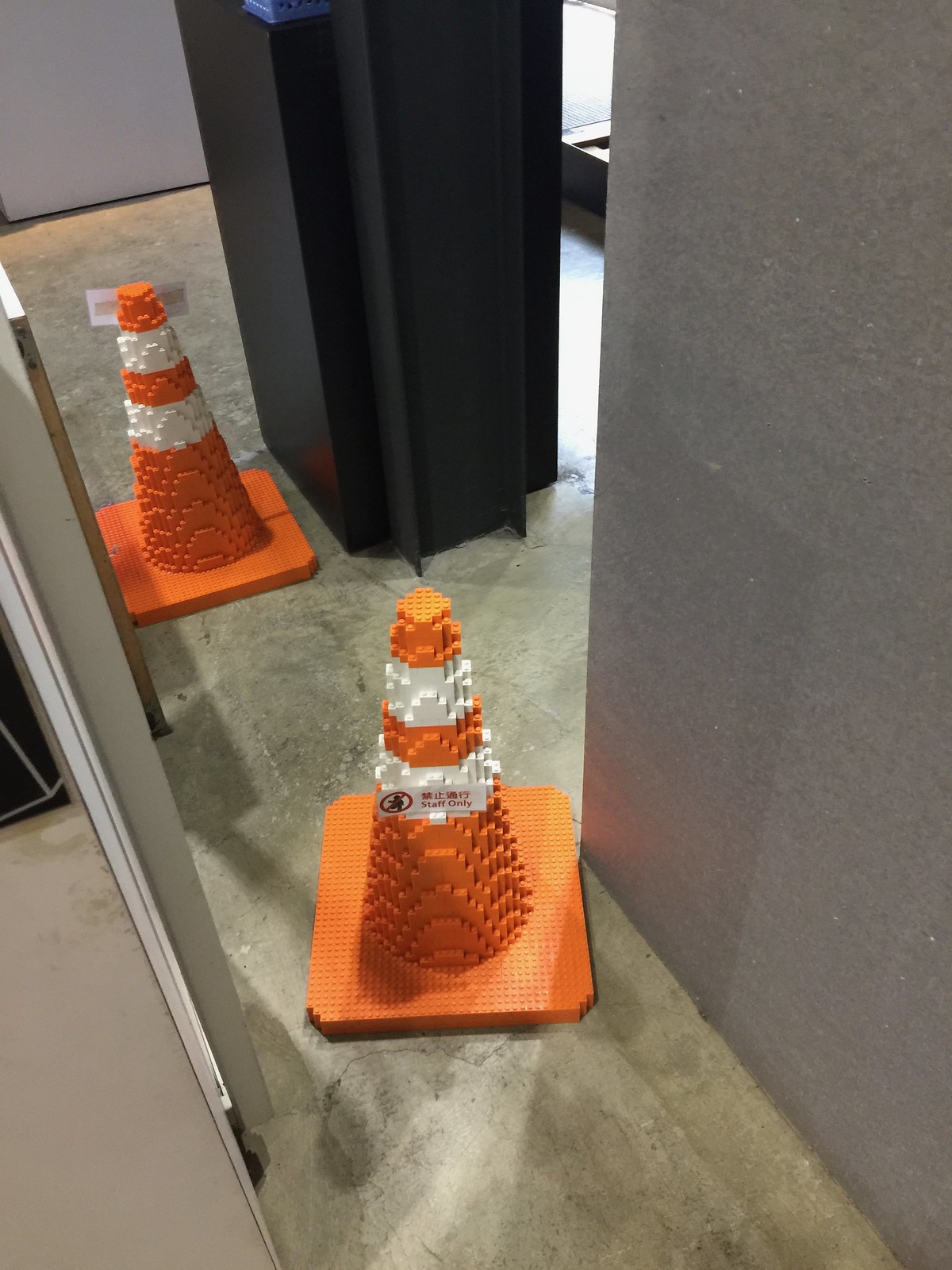The image depicts a virtual world scene set inside a building. To the left, there is a partial view of a gray table, with a small black square just off the top left corner of the frame. A light gray partition extends from the top left to the floor. The floor, which appears to be made of poured cement, slopes upward to the left and is adorned with pixelated, Lego-like traffic cones in orange and white colors. These cones resemble traditional caution cones, complete with alternating stripes and an orange cap, and one of them even bears a "staff only" tag. The floor leads to a dark gray wall and further along, to a corridor or hallway on an angle. In the center-right of the image, a large black column extends from the floor to beyond the top of the frame. The scene is detailed with an interplay of gray walls, the black pillar, and the intricately modeled Lego traffic cones positioned on the cement-like floor.